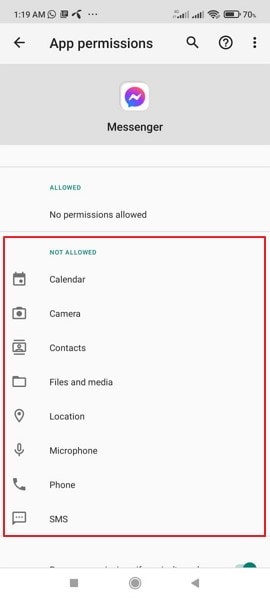A detailed descriptive caption for the provided image could be:

"A screenshot from a smartphone displaying the app permissions settings for the Facebook Messenger app. At the top of the screen, the status bar shows it is 1:19 a.m. on the left, with signal bars for cellular and Wi-Fi connectivity, and a battery icon indicating a 70% charge on the right. Below this status bar, a navigation bar contains an arrow pointing left for back navigation, a magnifying glass (search), a circular question mark (help), and three vertical dots (menu). The title 'App Permissions' is displayed prominently, followed by the Messenger app icon—a white chat bubble with blue, pink, and purple hues set against a white background. Beneath the icon, the permissions settings are divided into two sections: 'Allowed' and 'Not allowed.' The 'Allowed' section is empty, indicating that no permissions have been granted. The 'Not allowed' section, highlighted with a red border, lists various permissions that have not been granted, including Calendar, Camera, Contacts, Files and media, Location, Microphone, Phone, and SMS, each accompanied by respective icons. This detailed setting overview indicates a high level of restriction on the app’s access to the smartphone's resources."